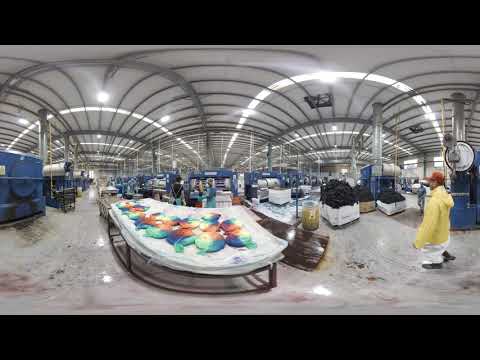The image depicts a large, well-lit warehouse or factory, characterized by a distinctive industrial ambiance with fluorescent lights and metal gray bars running across the ceiling. The spacious area is filled with long tables set up, which appear to house colorful, circular objects resembling tie-dye patterns, possibly flat-stuffed animals or unidentified items with extensions. Various carts and containers are scattered around, some containing unidentifiable black substances. There is a prominent figure in the scene, a factory worker dressed in a long yellow coat, white pants, boots, and an orange hat, who appears to be positioned to the right side of the image, near a white table and a golden bucket. The setting also features additional machinery and sections that might be workstations flanking the walls, contributing to the overall impression of a bustling production environment.